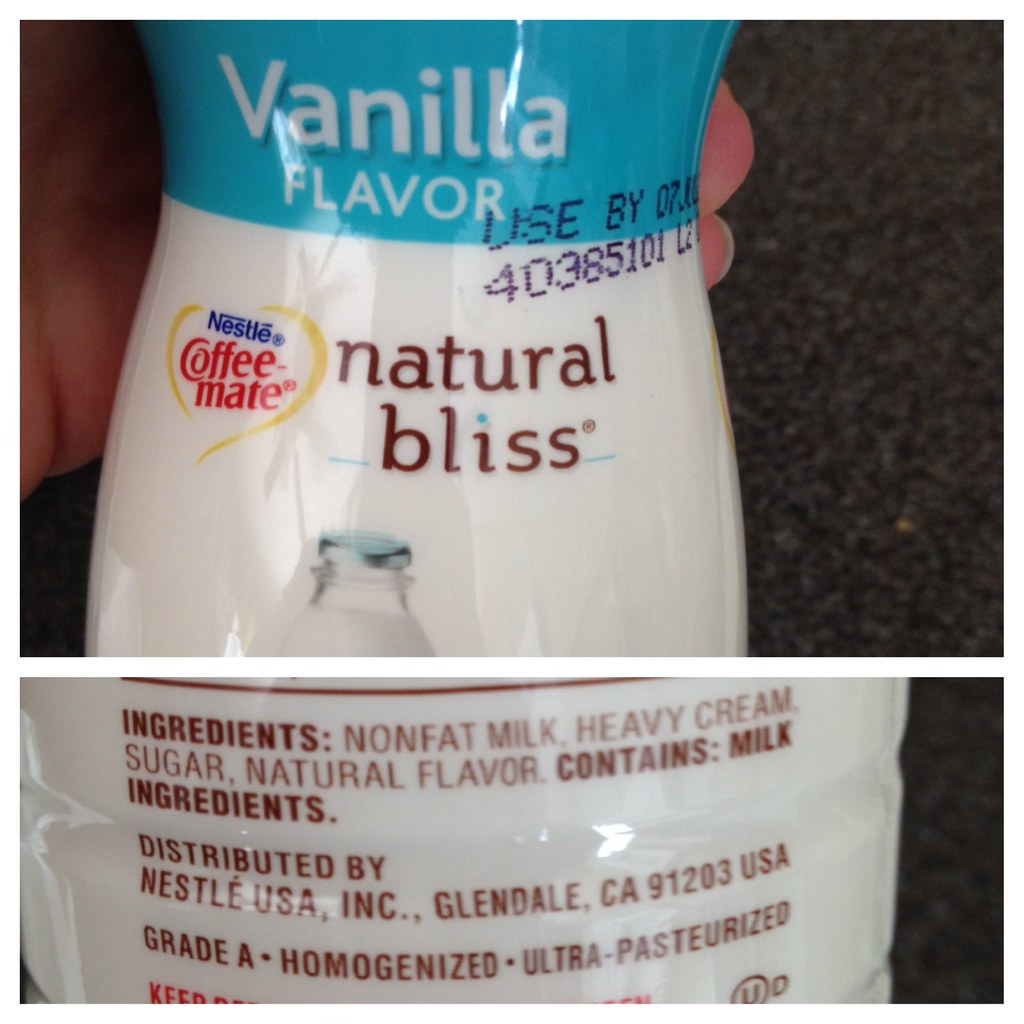The image consists of two photographs of a Nestle Coffee-mate creamer. The top photograph prominently displays the front of the creamer bottle, which features a vanilla flavor. The bottle has a light blue background, with the main section being white. The front label highlights that the creamer is "Naturally Gloss." The Nestle Coffee-mate brand name is clearly visible. The bottom photograph showcases the back label of the bottle, detailing the ingredients, which include nonfat milk, heavy cream, sugar, and natural flavors. The product is manufactured by Nestlé USA, Inc., located in Glendale, California.